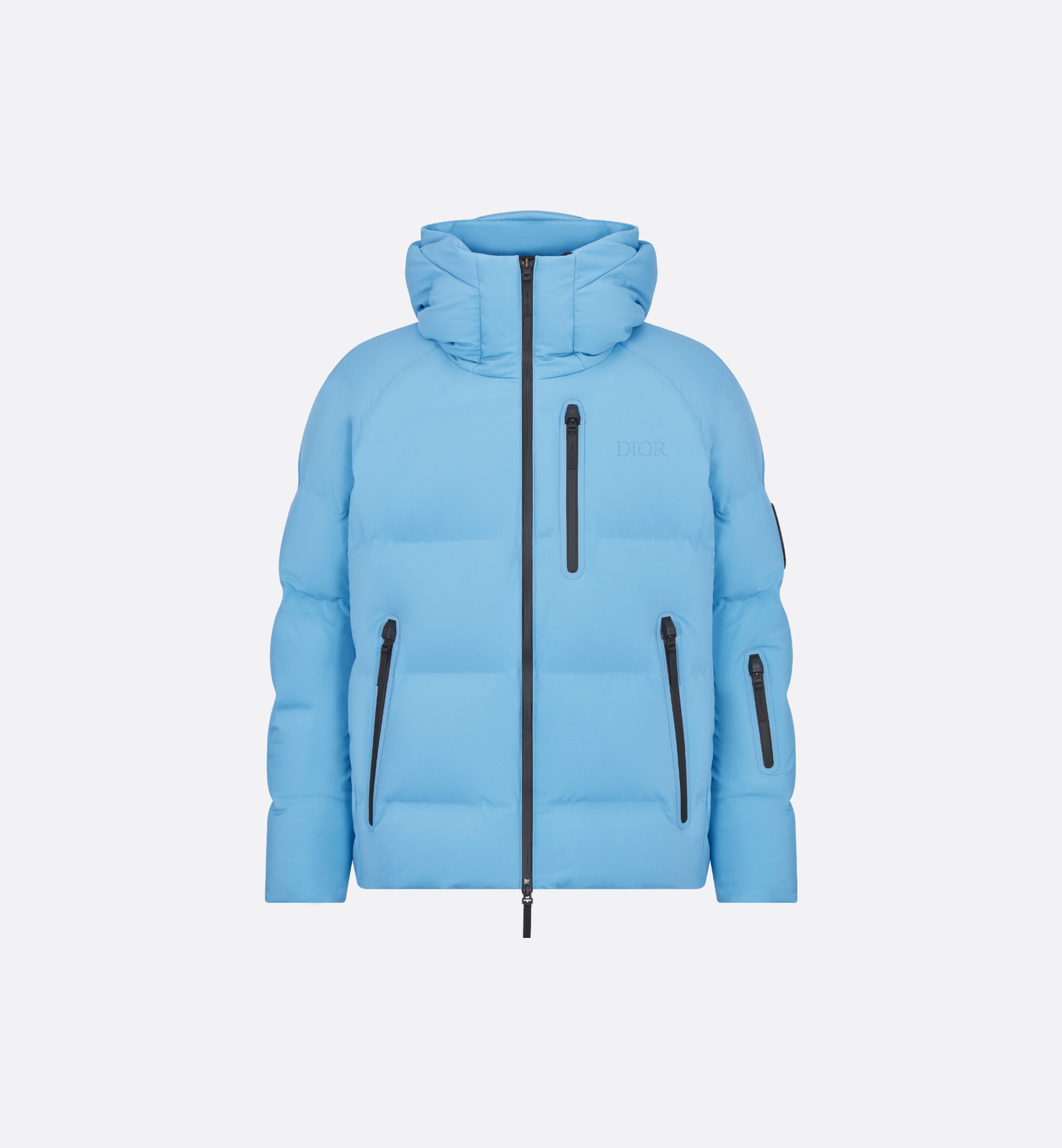The photograph showcases a light blue puffer jacket suspended in mid-air against a solid, very light gray background. The jacket features a high neck and multiple dark gray to black zippers: one down the middle, one on the chest, one on either side of the waist, and an additional zipper pocket on the left sleeve. The material appears puffy, indicating its suitability for cold weather activities like skiing. The word "D.I.O.R." is inscribed on the top left chest area of the jacket. The clean and minimalistic composition suggests that this image is likely intended for showcasing the jacket as a product, perhaps for online retail.